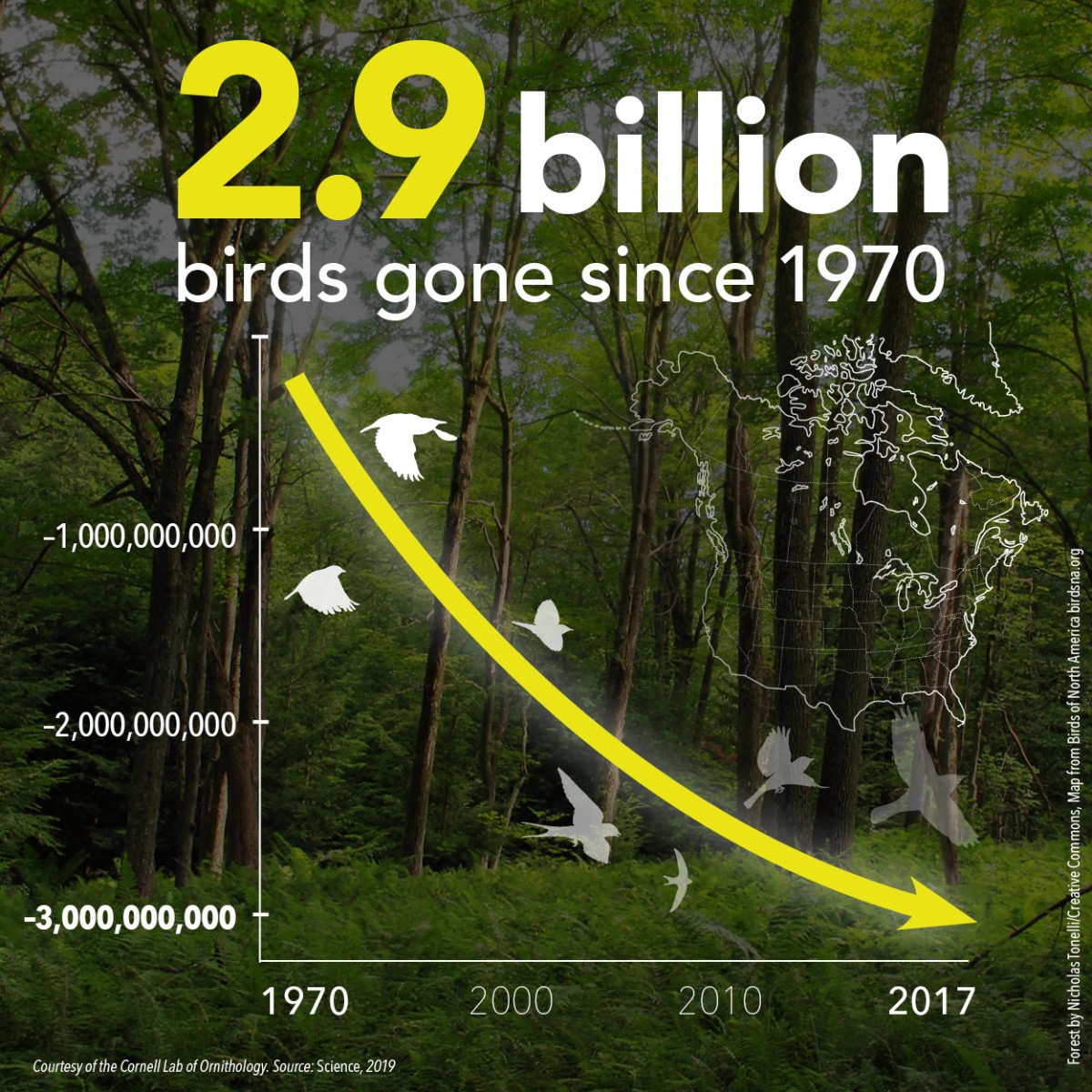This detailed informational graphic poster highlights the staggering decline of bird populations in North America since 1970 against a forest backdrop with lush trees and tall green brush. Dominating the top portion in bold yellow and white text, the headline starkly states: "2.9 billion birds gone since 1970." Prominently featured is a large, transparent graph which is overlaid with an arrow that descends from left to right, symbolizing the consistent reduction in bird numbers over the years. The vertical axis marks intervals at 1, 2, and 3 million birds, while the horizontal axis spans from 1970 to 2017, further divided into key years: 1970, 2000, 2010, and 2017. Interspersed along the downward arrow are various white birds in flight, representing species like pheasants and grouse. A white, transparent graphic depicting North America occupies the top right corner, reinforcing the geographic context of the data.